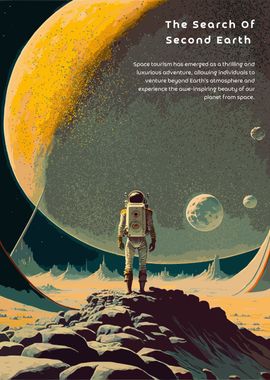This detailed image appears to be the cover of a science fiction novel entitled "The Search of Second Earth." Dominating the top half is a large gas giant, somewhat like Jupiter or Saturn, with a distinct appearance: a dark right side and a yellowish left side due to lighting from the left. Three smaller moons, visible in the bottom right in front of the gas giant, suggest a complex planetary system. An astronaut in a white space suit, complete with space gear and a white equipment box on his back, stands atop a mound of gray rocks, his back turned towards the observer as he gazes at the expansive celestial scene. The cover features a block of text beneath the title describing space tourism as a thrilling and luxurious adventure, highlighting the awe-inspiring beauty of Earth from space. Though the text is somewhat blurred and challenging to read, it underscores the theme of exploration beyond Earth's atmosphere. There is no atmosphere visible around the astronaut, emphasizing the barren terrain, presumably on one of the gas giant’s moons.